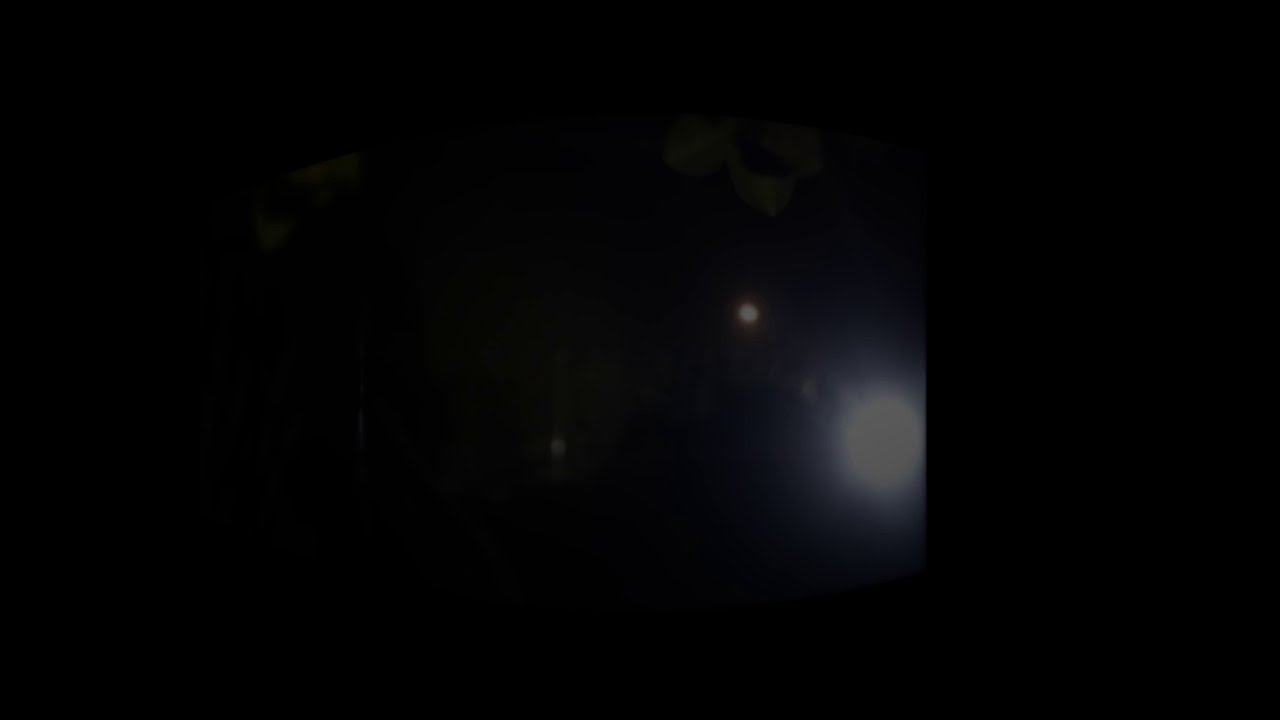The image is a dark, portrait-oriented photograph with prominent black bars on the left and right sides, creating a narrow, vertical view in the center. The main visual elements consist of a bright yellow light positioned in the bottom right corner, roughly a third of the way from the edge. Just above and slightly to the left of this large light, there is a smaller, dimmer ball of light. Both lights rest on a completely solid black background, creating the impression of viewing distant lights at night.

In the upper left and right corners of the image, faint traces of green leaves are visible, suggesting an outdoor setting, possibly near a street with a pole and streetlight. Additionally, there is a soft, ambient glow, like an amber-colored street lamp, and the possibility of a reflective surface indicating a ceiling fan indoors is noted—although this may also be a reflection of an outdoor scene. Overall, the photograph captures a minimalistic nighttime scene with a few key light sources against a stark black backdrop.